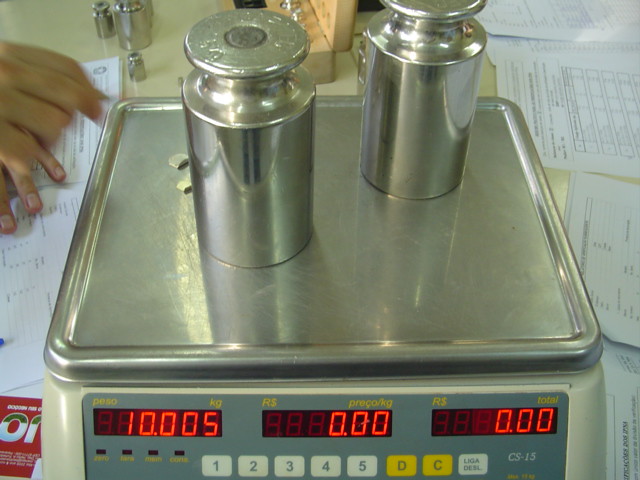This image features a sophisticated weighing machine with a silver, square-shaped design, supported at its four corners. On top of the machine, there are two cylindrical bottles with intricately shaped tops that taper inward before widening again and are capped with silver lids featuring darker silver centers. One bottle is positioned near the top right, partially obscuring the view of the second bottle beneath it, which also has a silver lid.

The front panel of the machine is adorned with a grey background and includes multiple digital displays with red-lit numbers. The first opening shows "10.005 kgs," the second displays "000," and the third reads "0.00." Below these displays, there is a series of white buttons numbered 1 through 5, alongside yellow-labeled buttons inscribed with letters like "d" and "c." There is an additional white button with illegible text.

On the right side of the image, some white papers are visible, featuring diagrams and black text. Similar papers are also placed on the left of the machine. A person's hands are seen entering the frame, indicating interaction with the device.